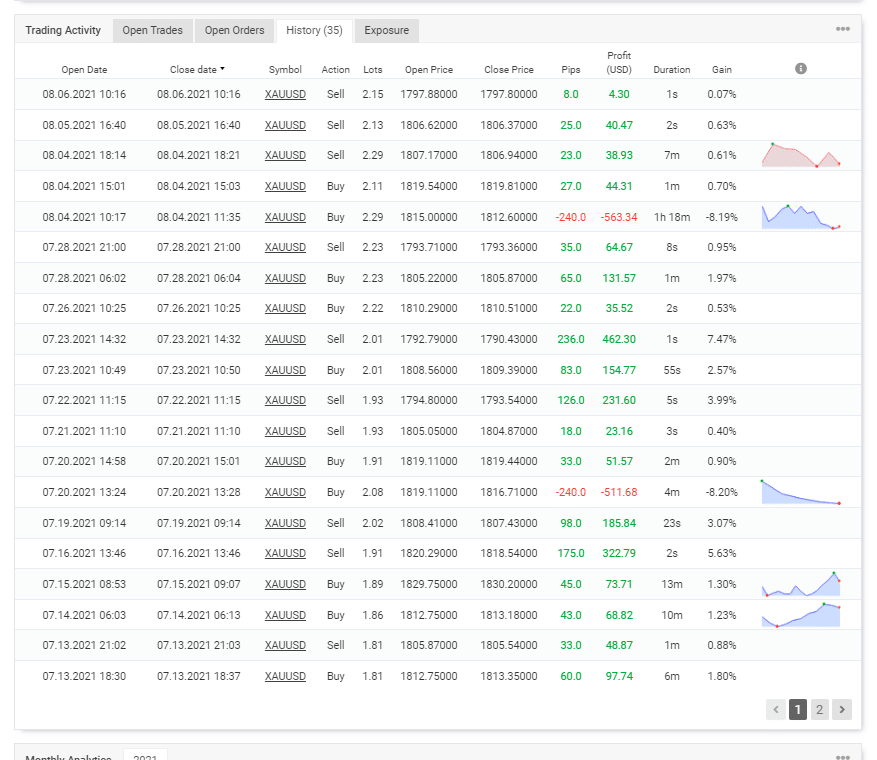The image showcases a detailed stock exchange table set against a primarily white background. At the top of the interface, there is a header with a light gray background and a medium gray border, featuring several tabs labeled: **Trading Activity, Open Trades, Open Orders, History,** and **Exposure**. The **History** tab is prominently selected, indicated by its white background, blending into the main page, and a notation in parentheses stating (35) next to it.

The table columns are titled in a simple format: **Open Date, Close Date** (with a downward arrowhead suggesting a dropdown menu), **Symbol, Action, Lots, Open Price, Close Price, Pips, Profit (USD), Duration**, and **Gain**. To the right of these columns, there is a gray-filled circle with an italicized lowercase "i" representing additional information. In the upper right corner of the header, three gray dots hint at more options accessible via a click.

The first row of the table is highlighted with a light bluish-gray background. In a basic, small sans-serif black font, the data is populated as follows:
- **Open Date**: 08.06.25
- **Close Date**: 08.06.2021 10:16
- **Symbol**: XAUUSD (underlined)
- **Action**: Sell
- **Lots**: 2.15 
- **Open Price**: 1797.88000
- **Close Price**: 1797.80000
- **Pips**: 8.0 (in green)
- **Profit (USD)**: 4.30 (in green)
- **Duration**: 1S (in black)
- **Gain**: 0.07% (in black)

Each element is meticulously designed to provide clear, concise information about the trading activities recorded in the history tab.